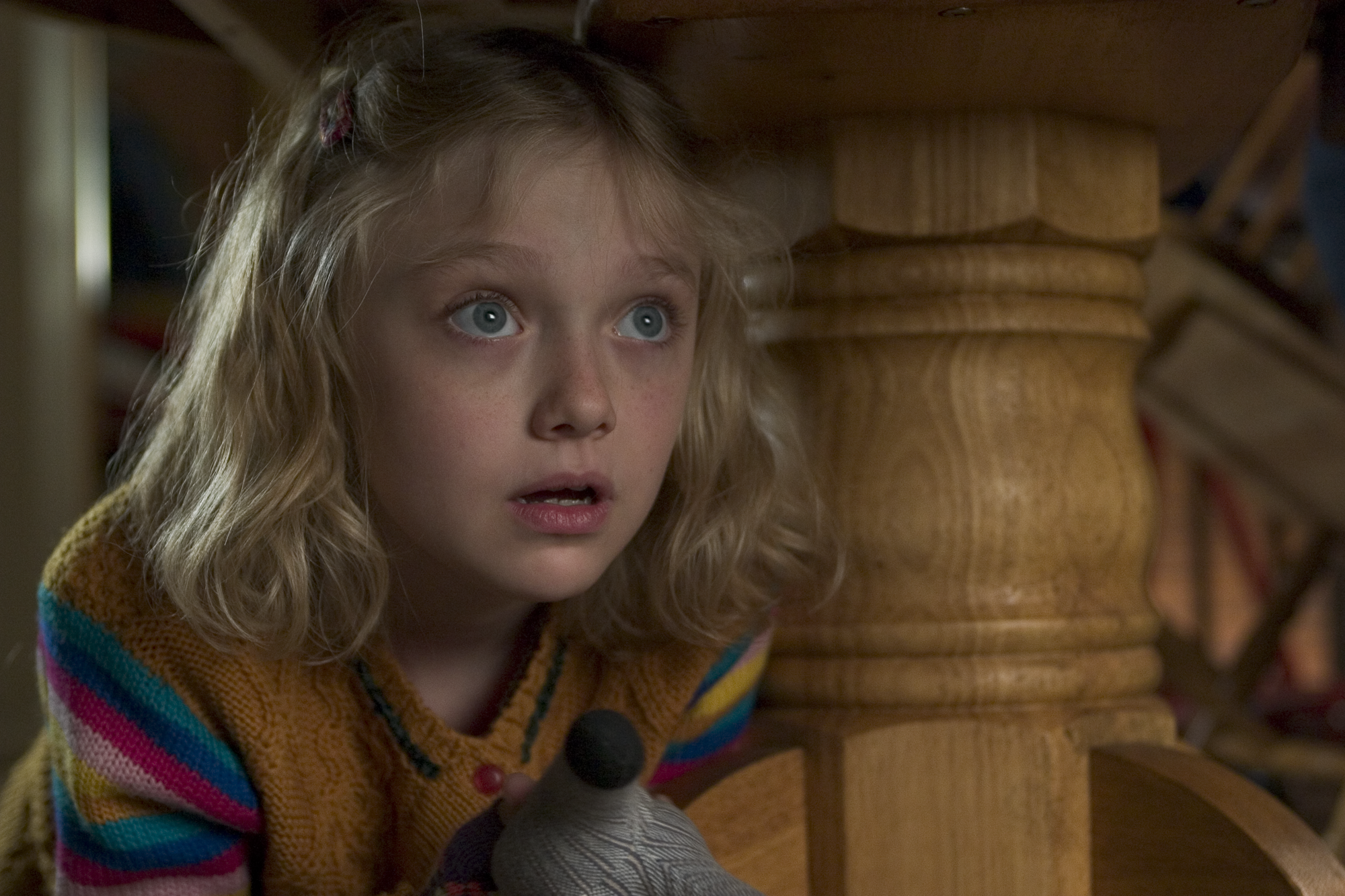This photograph captures a young child, probably a girl in the age range of 8 to 10 years, with long blonde hair falling to around shoulder length. She has striking blue eyes that are wide and full of a mix of curiosity and surprise as she gazes towards the top right corner of the image. The child, who appears somewhat startled with her mouth slightly open, is crouched underneath a light brown wooden table with a thick single leg. Illuminated by light coming from the upper left that accentuates her hair, she clutches a gray stuffed animal with a black dot, which could be a dog or a mouse. She is dressed in a gold-colored button-up sweater with a blue line along the collar, and sleeves adorned with colorful stripes in blue, light blue, purple, pink, and yellow. The overall composition, with her expression and position under the table, evokes a sense of a scene pulled straight from a movie still.